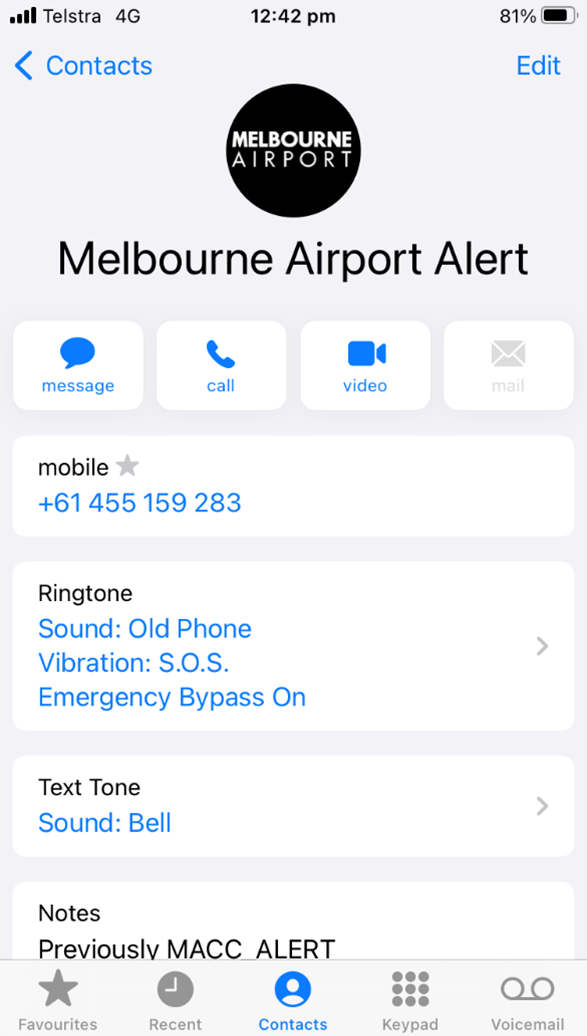This image depicts the contact page of a smartphone screen, presumably showing contact details for "Melbourne Airport." At the very top left of the screen, the mobile carrier "Telstra" is visible with four bars of signal strength, indicating strong connectivity. To the right, the network is labeled as "4G," and the current time, displayed in bold black text, reads "12:42." Next to the time, the battery icon shows 81% charge remaining.

Below this status bar, an "Edit" button in blue is present. The header shows "Contacts" with a back arrow on the left. Below the header, "Melbourne" is displayed within a black circle, followed by "Melbourne Airport" in bold text.

The contact page contains four interactive buttons with rounded corners: "Message" (with a blue message icon), "Call," "Video," and "Mail" (shown in gray).

Further down, the contact details include a mobile number formatted as +61 445 159 283. Notable settings include the ringtone labeled "Old Phone," vibration set to "SOS," and emergency bypass turned on (indicated in blue text). The ringtone selection is highlighted in black text.

The text tone is set to "Sound Bell." At the bottom of the screen, a section for notes mentions a previous entry labeled "MACC."